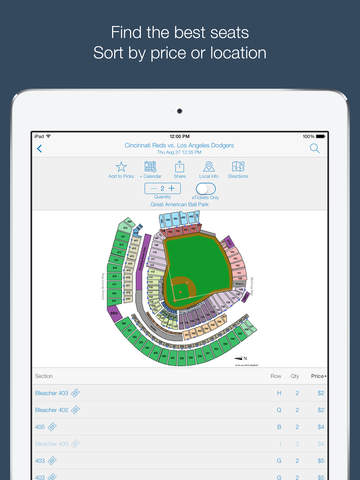This image is a screenshot from a ticket sales app, displaying a page with a dark blue background. At the top center, white text reads, "Find the best seats - sort by price or location." Below this header, a white iPad is prominently featured, showing the app's interface. The iPad screen displays a stadium photo, centrally positioned, with a list of available tickets underneath. The image is cropped, cutting off the bottom half of the iPad, and no branding is visible. The app page specifically references a Dodgers game, with the Cincinnati Reds playing against the Los Angeles Dodgers.